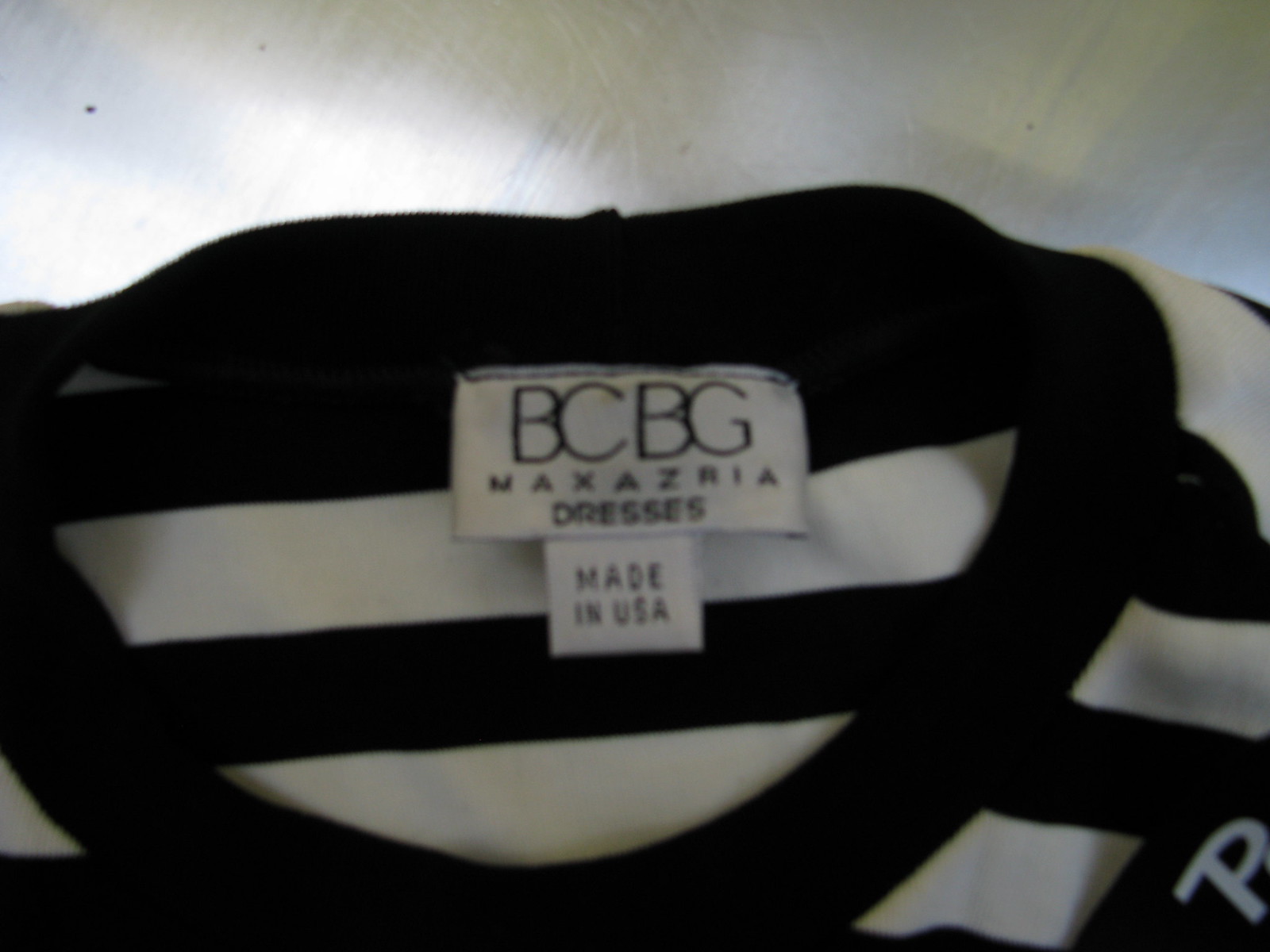The image shows a close-up, slightly out-of-focus view of the inside collar of a black and white striped t-shirt with a black collar. The tag inside the collar is white with black lettering, stating "BCBG Max Azria Dresses." Below this tag, there's another smaller white tag that reads "Made in USA." The shot includes a bit of the wall behind the shirt and captures part of the shirt's pattern, which consists of alternating black and white lines. In the bottom right corner of the image, a portion of a straight black line with a "P" is visible, but it doesn't contribute to the main focus on the tags and collar detail of the t-shirt.